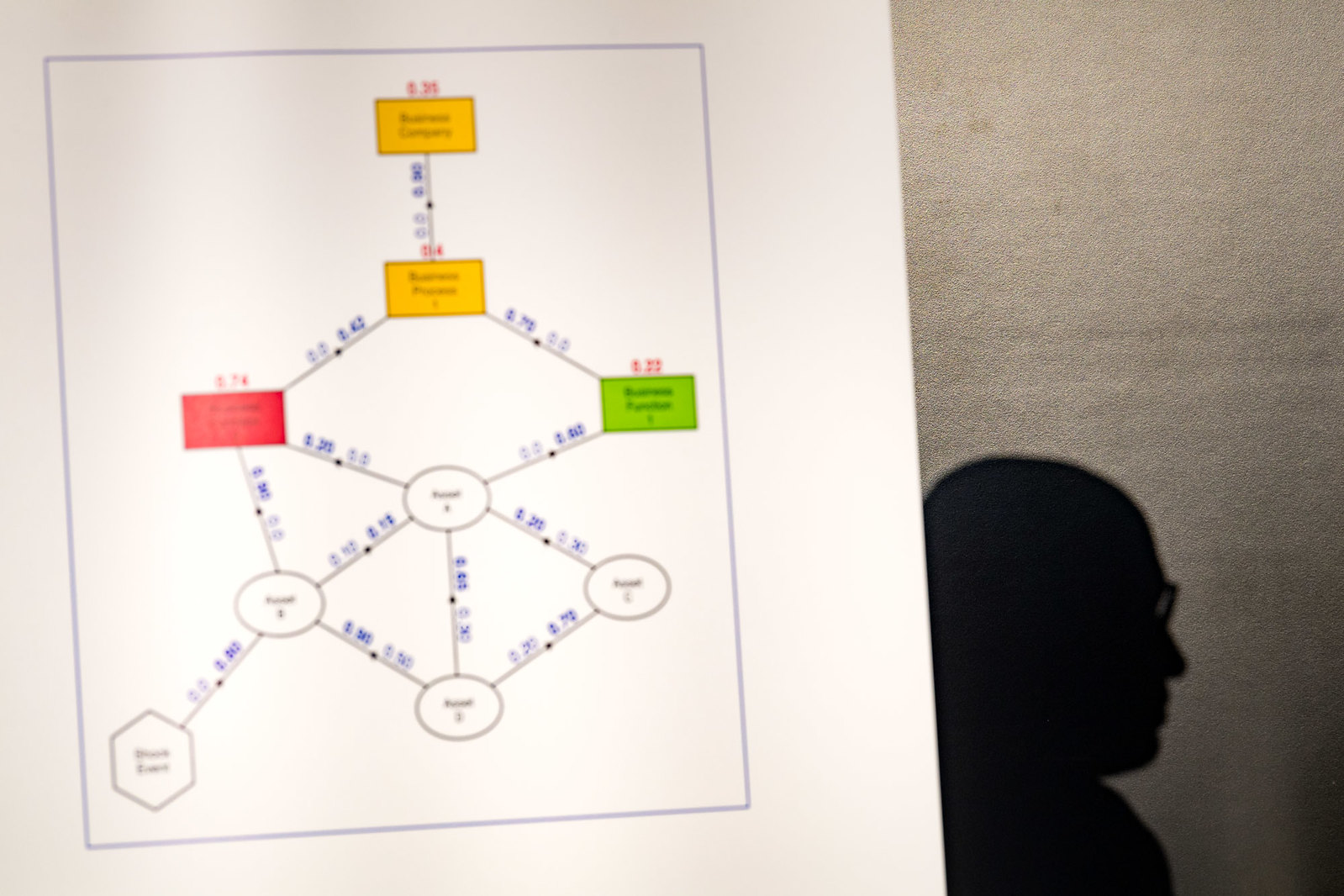The photograph captures a scientific diagram that, unfortunately, is too blurry to discern the specific text within. Central to the diagram are two yellow boxes connected sequentially, where the second yellow box branches into a red box on the left and a green box on the right. These boxes then lead into a central white oval shape, which subsequently connects to three additional oval shapes. One of these ovals, positioned towards the left of the image, transitions into a hexagonal shape. Each geometric figure in the diagram contains letters, and the connecting lines display numbers or mathematical equations in blue ink.

A thin blue line frames the entire diagram, which is situated on a white poster board or sheet. In the background, there is a shadow or silhouette of a bald man wearing thick-rimmed glasses, projected onto what appears to be a concrete wall. This shadow is slightly fuzzy around its edges, suggesting a diffuse light source. The poster is illuminated by a bright light originating from the bottom left corner, off-screen.